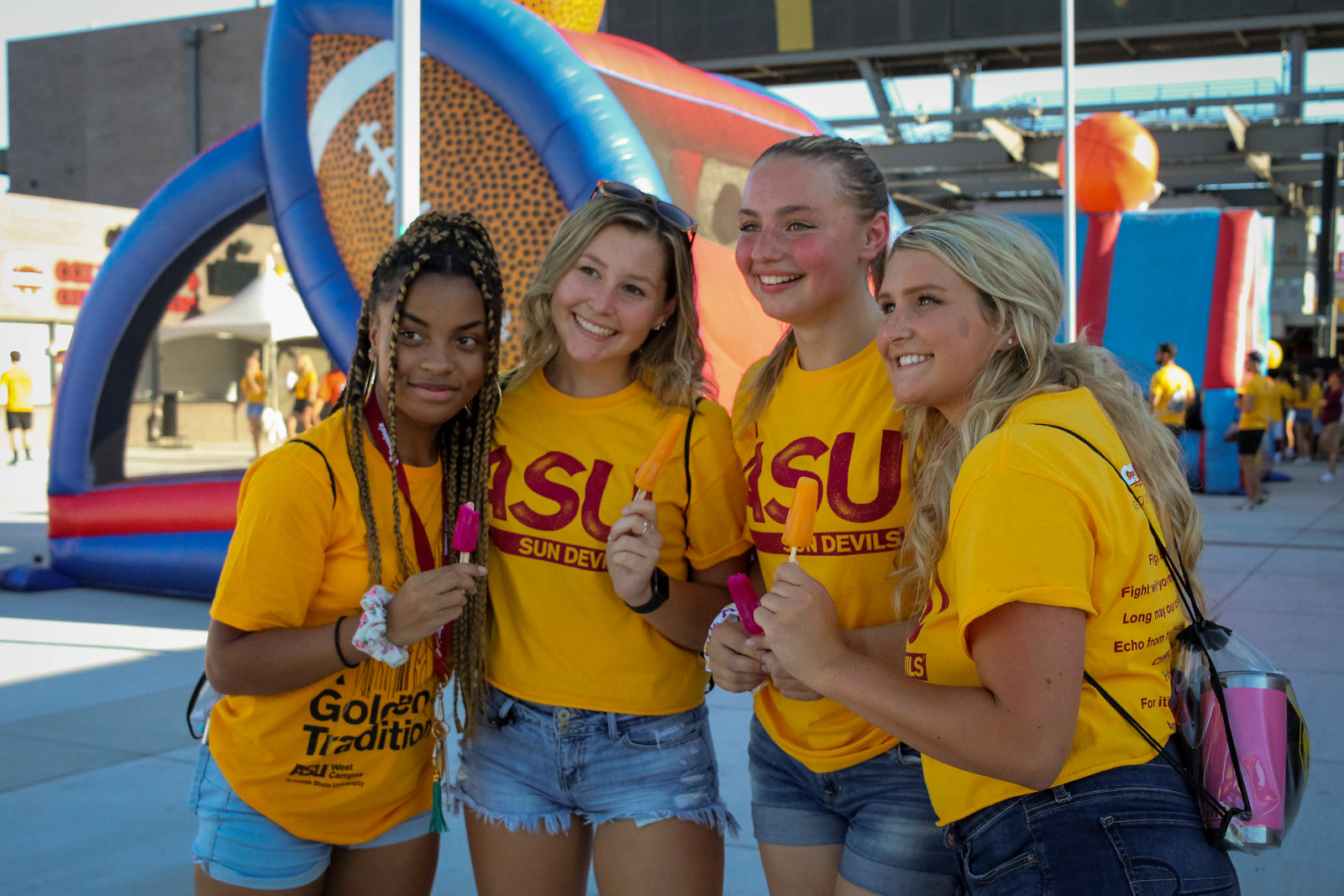The image captures a vibrant and sunny day at an outdoor festival, with four college-aged girls from Arizona State University (ASU) joyfully posing together. Three of the girls are white with blonde hair, while one is black with brownish-blonde hair. They're all wearing bright yellow ASU Sun Devils t-shirts, some adorned with red lettering and the words "Sun Devils" or “Golden Tradition” in black. Each girl is holding a popsicle and smiling radiantly, suggesting they've been enjoying a fun-filled day under the sun. Clad in jean shorts, they embody the carefree spirit of summer. Behind them, the scene is lively with inflatable games, bouncy castles, and slides, indicating a bustling and family-friendly festival atmosphere. One girl has a clear purse slung behind her, with a water bottle and a few other items visible inside. The backdrop and their happy expressions exude a sense of camaraderie and enjoyment.